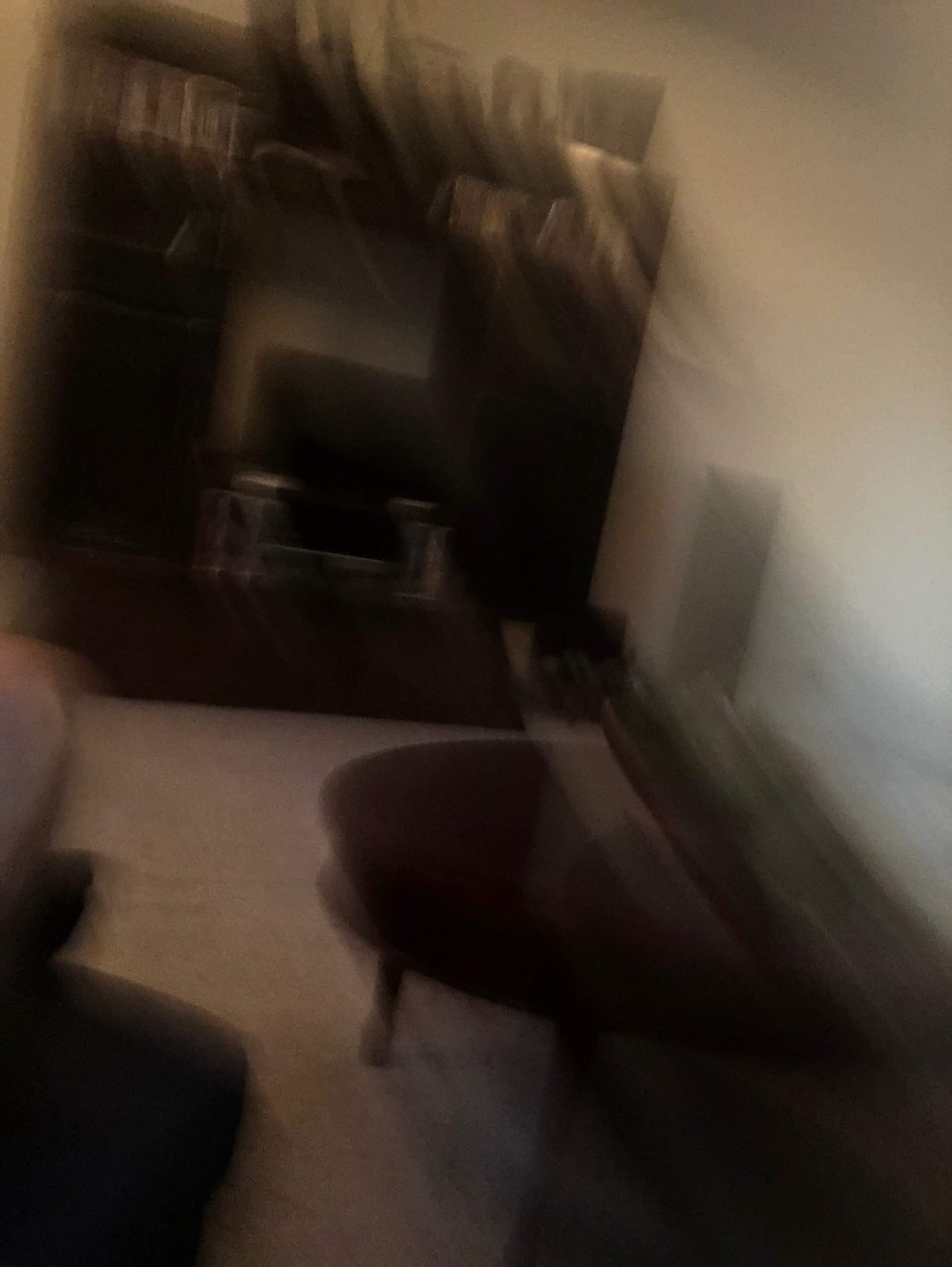This photograph captures a living space, but it is very blurry due to apparent camera motion, causing a streak effect diagonally down towards the right. Despite the blurriness, several features are discernible. There is an entertainment stand with a thin black television, surrounded by white walls. The entertainment stand, characterized by its brown hue, seems to be flanked by bookshelf-style sections that might house DVDs, CDs, or video games, though specifics are obscured. Above the stand, a mantle holds several indistinct picture frames. 

A brown, round wooden coffee table with cylindrical legs occupies the foreground, featuring a plant whose green foliage streaks downward diagonally in the image. The room includes a white or light gray carpet. To the left, parts of a tan or dark gray couch or chair are visible, and a possible glimpse of a person’s leg in dark pants can be seen. There’s also a little rectangular area near the entertainment stand, possibly a small doorway, adding to the room’s intriguing yet unclear layout. The overall image has a sepia-toned appearance, further enhancing the brown hues throughout.